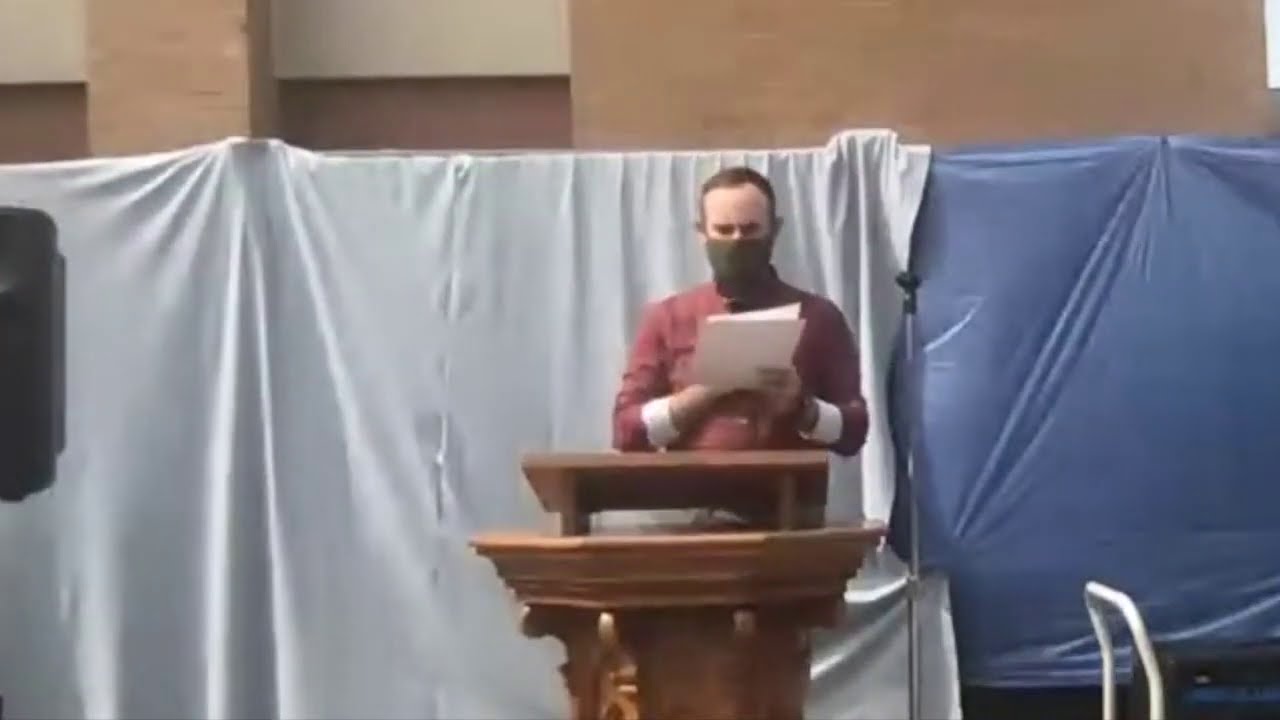The image depicts a man, likely a pastor or preacher, standing prominently at an ornate wooden lectern in the center of a horizontal rectangular room. He is dressed in a light burgundy dress shirt with distinctive white cuffs and is wearing a black mask. The man's thinning brown hair is visible as he holds some white pieces of paper, appearing to read from them. The lectern, made from brown wood, features detailed carvings, ornate ledges, and curved pillars running up the sides, with a stand on the top for holding papers and books. To his right, a microphone stand is visible, although the microphone is missing.

Behind the man, the wall is draped with large sheets in different colors; the left and center sheets are white, while the right sheet is blue. These cloths obscure most of the underlying wall, but some parts of the structure can be seen, including a recessed brown section and a white section that protrudes slightly more than the rest. Additionally, there is a brown brick-like pillar and more of the recessed brown wall with the same white protrusion on top. On the left, there's a partial view of a black speaker, and at the bottom right corner, the white handle of a cart is visible. The overall backdrop suggests a makeshift or temporary setup, possibly for an impromptu gathering or event.